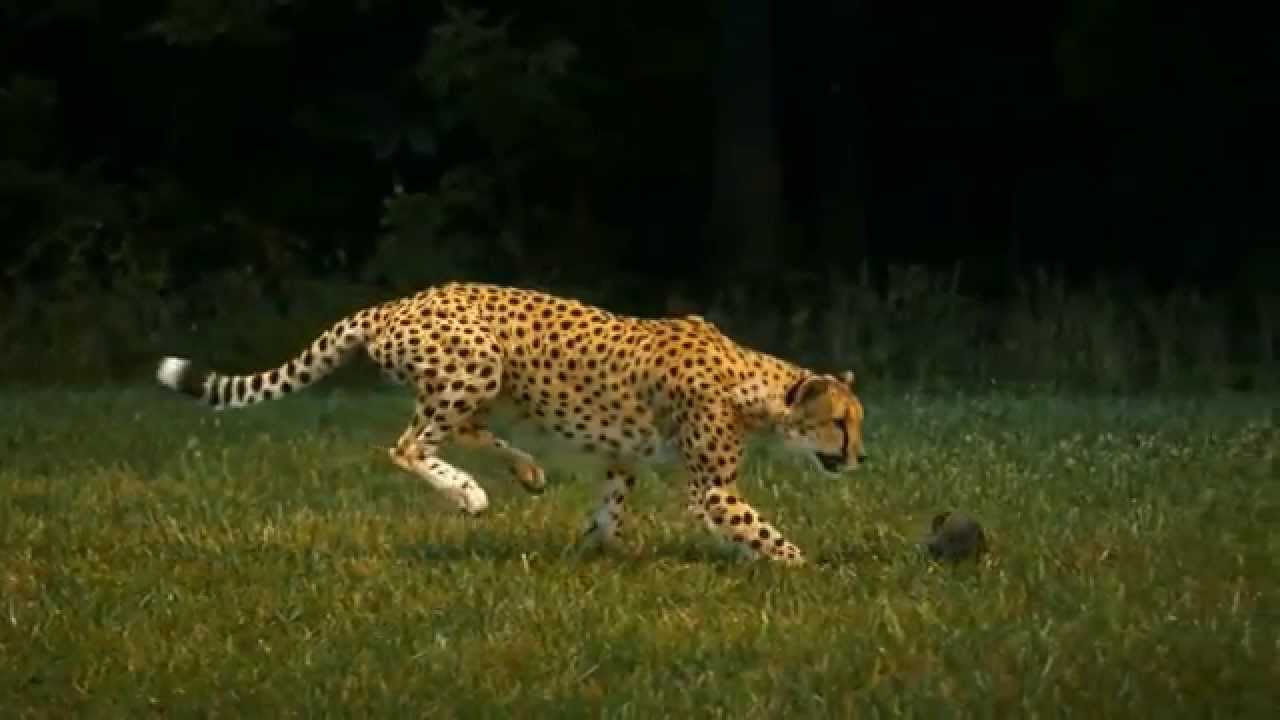This is a photograph capturing a side view of a predatory feline, which could be either a leopard or a cheetah, in a dynamic, nighttime setting. The creature, characterized by its black spots and a white-tipped tail, is caught in motion, seemingly about to catch something as it strides through grass that is predominantly green with patches of brown. The clarity of the image is compromised, making the animal appear blurred. The ground is spotted with a black stone towards which the feline seems to be gazing. The scene is enveloped in darkness, with a completely black sky and indistinct outlines of distant bushes and trees.